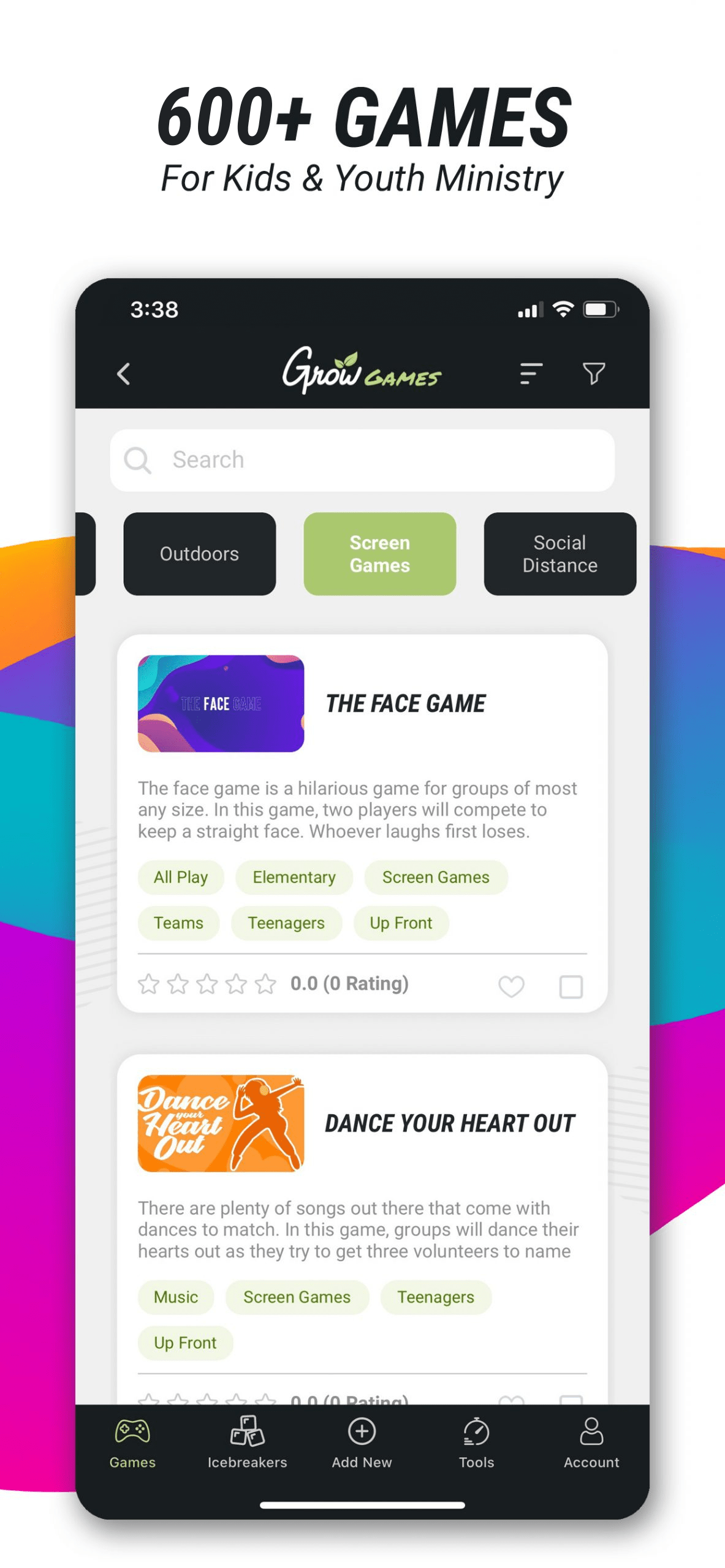The image is a screenshot of a smartphone displaying an app titled "Grow Games" at the top, with a header that reads "600+ games for kids and youth ministry" in black text on a white background. The screen shows information organized in a user-friendly interface. At the very top, within a black border, is the current time of 3:38, signal strength with three bars out of four, and a battery level at around 90%.

Beneath this, there is a search bar followed by three rectangular buttons labeled "Outdoors," "Screen Games," and "Social Distance." These buttons help users navigate the app's categories. Below the buttons are two featured games.

The first game is called "The Face Game," with a dark blue icon. The description says, "The Face Game is a hilarious game for groups of most any size. In this game, two players will compete to keep a straight face. Whoever laughs first loses." This section also includes multiple buttons for further actions and a star rating system.

The second game, "Dance Your Heart Out," has an orange-themed icon and features a silhouette of a dancing woman. Its description reads, "There are plenty of songs out there that come with dances to match. In this game, groups will dance their hearts out as they try to get three volunteers to name the moves." This game also includes several buttons for interaction.

At the bottom of the screen, there are menu options labeled "Games," "Icebreakers," "Add New," "Tools," and "Account," with "Games" highlighted in light green.

The background of the image is a colorful ad featuring pink, turquoise, and purple hues, providing a vibrant context to the displayed app screen.